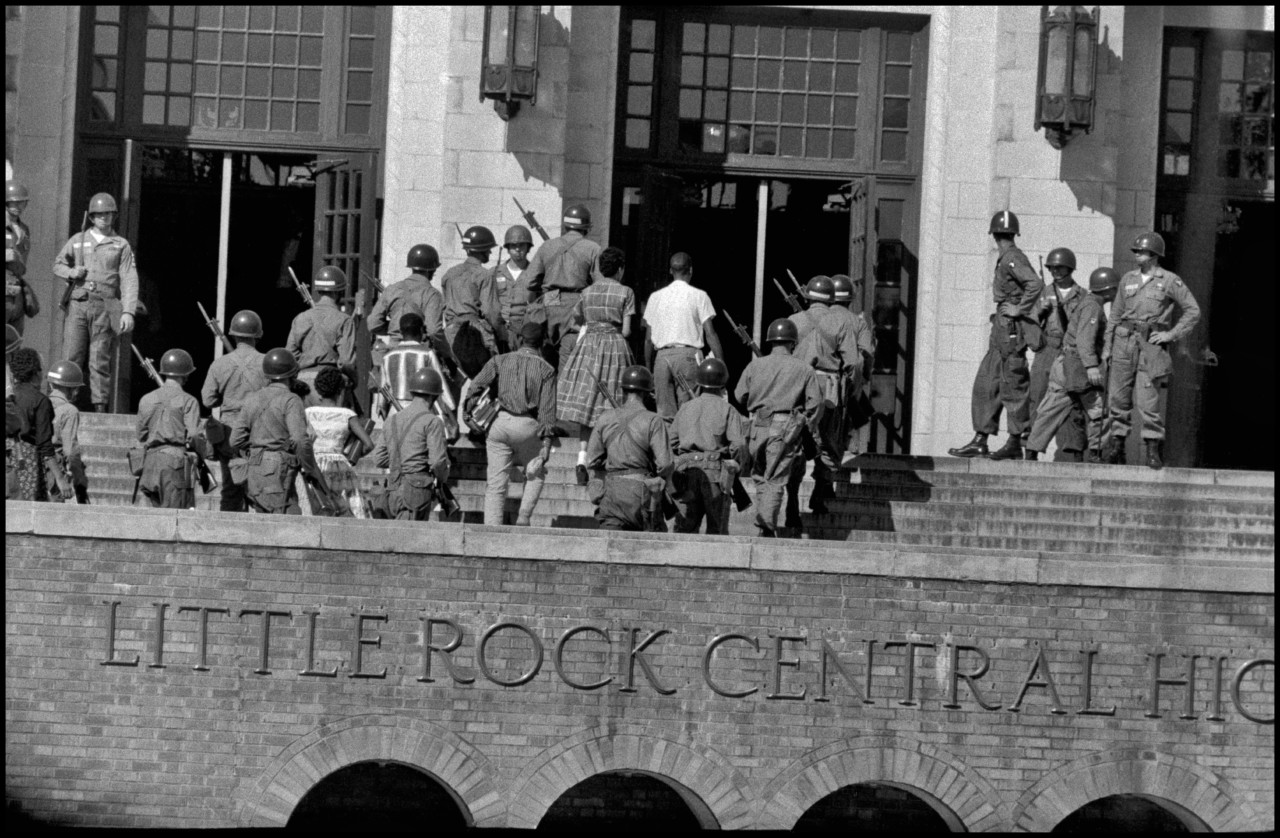This is a powerful black and white archival photograph depicting a pivotal moment in American history – the desegregation of Little Rock Central High School in the 1950s or 1960s. The image captures a tense scene with a brick or stone facade building in the background, clearly marked "Little Rock Central High." The doors of the old, stately school building become the stage for this historic event. Centered in the photo are five to six young Black students, solemnly walking up the steps, escorted by teachers and flanked by members of the National Guard. The soldiers, clad in what was considered riot gear of the time, complete with helmets and bayonet-fixed rifles, form a protective yet imposing barrier. The National Guard, deployed by the governor to prevent these students from entering, stand vigilant at the school's entrance, ready as if for combat. Part of the soldiers stand aside, observing the students' courageous steps towards the school, embodying both the confrontation and resilience of the era's civil rights movement. This image poignantly captures the intense opposition to desegregation and the bravery of the students who dared to cross those boundaries.